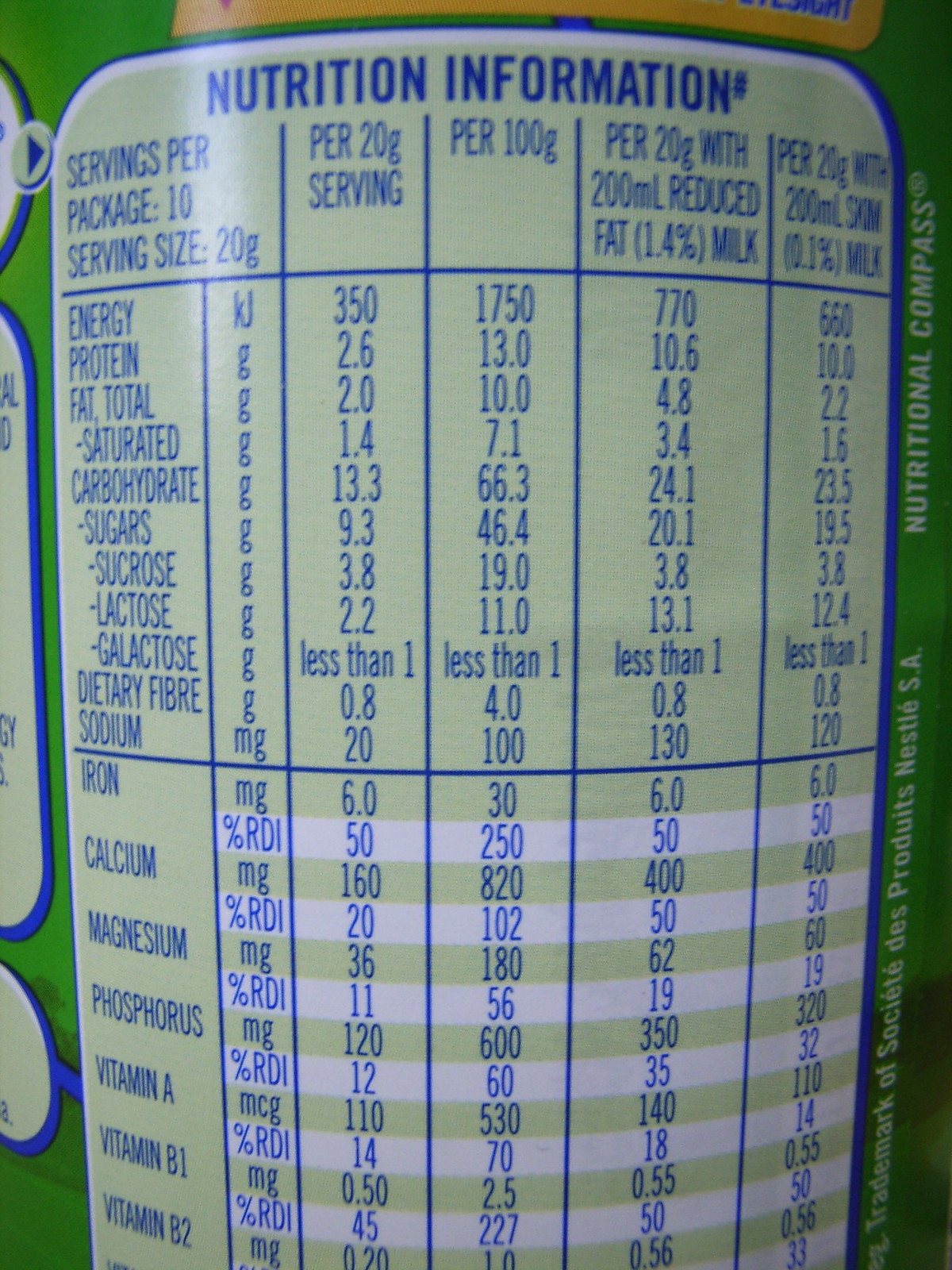This vertically rectangular image showcases a close-up of the nutrition information panel on the side of a Nestle product bottle. The panel, bordered in green, features a background that transitions from light green at the top to white stripes towards the bottom. The information is printed in blue and details comprehensive nutritional data. At the top, the title reads "Nutrition Information," followed by key metrics including servings per package (10) and serving size (20 grams). It delineates values for energy, protein, fats (total and saturated), carbohydrates (including sugars like sucrose, lactose, and galactose), dietary fiber, and sodium. A blue line separates these general nutrients from the listed minerals and vitamins such as iron, calcium, magnesium, phosphorus, vitamin A, vitamin B1, and vitamin B2. The data is provided per 20 grams and per 100 grams of the product, and an additional column states values per 20 grams with 200 milliliters of a reduced component. The information is meticulously arranged in rows that quantify the grams and percentage of Recommended Dietary Intake (RDI) for each nutrient.